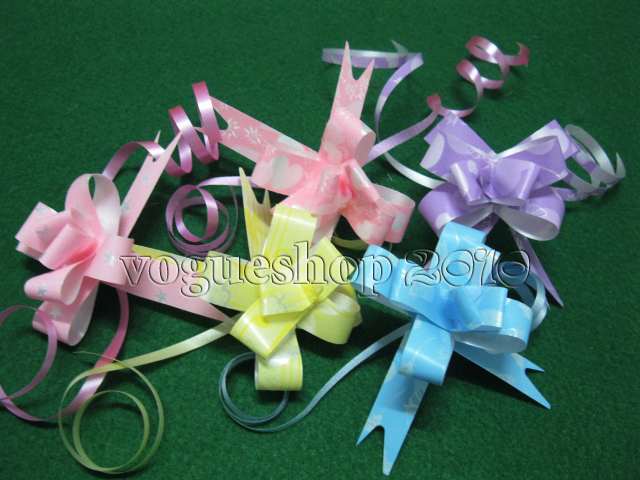The colour photograph showcases an assortment of brightly coloured gift ribbons, including shades of pink, purple, yellow, and light blue, artistically scattered and partially overlaid on a green felt background reminiscent of a billiards table. The ribbons, some of which feature pre-tied bows with cascading, curly ends, appear to be made of plastic. These decorative bows, traditionally used to finish gift wrapping, are prominently arranged to highlight their array of vibrant colors and intricate designs. Centrally placed, yet slightly below the middle of the image, is a watermark that reads "Vogue Shop 2010" in a see-through and etched style, suggesting this image is a promotional advertisement for the brand's ribbon products.